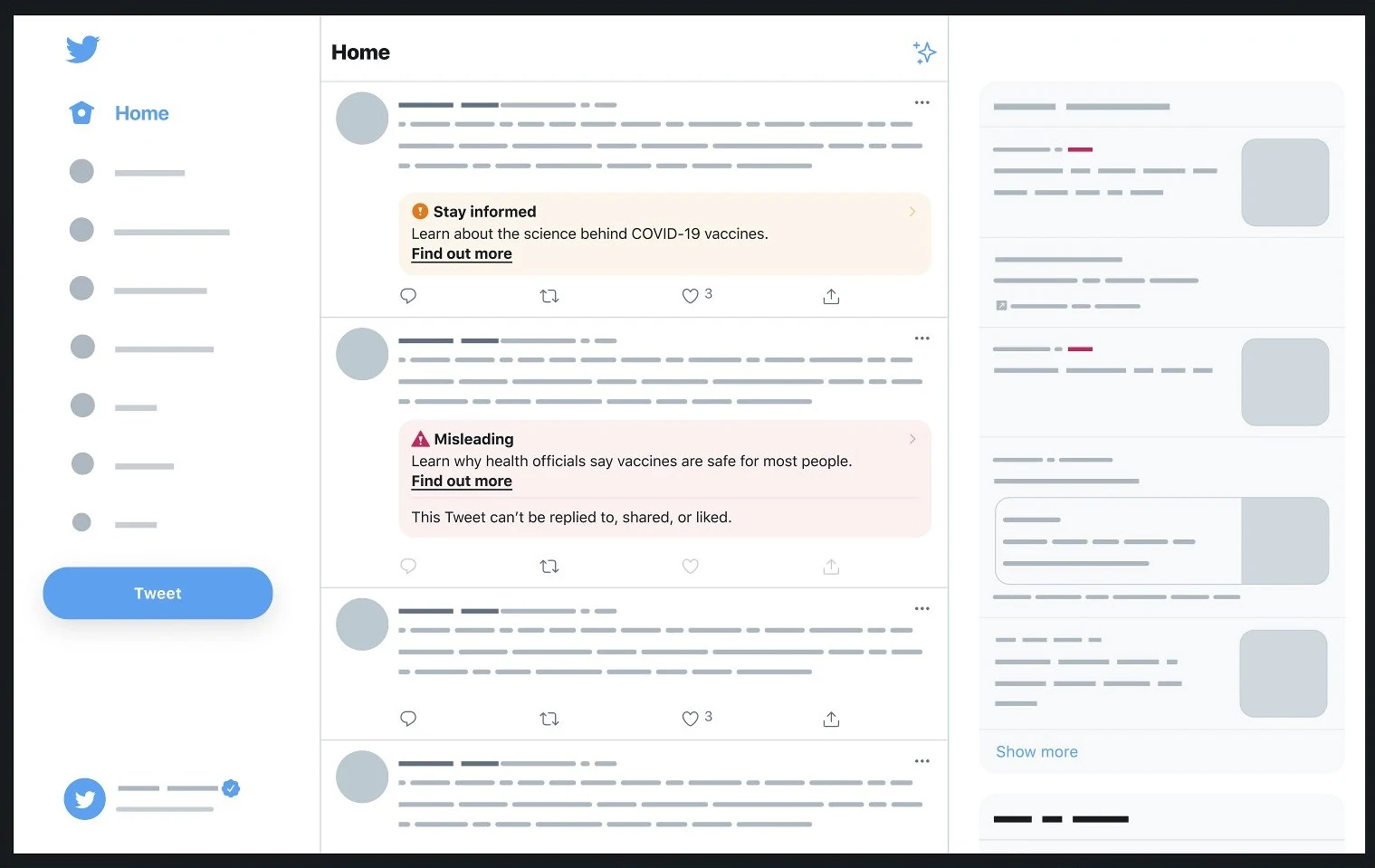The image depicts a mock-up of a Twitter interface with several distinct elements and alerts. 

On the left-hand side of the screen, there is an unpopulated bezel featuring grey lines and grey circles. At the top of this bezel, the Twitter logo is displayed as a blue bird. Directly beneath the bird icon is a house symbol, next to which the word "Home" is written in blue text. Towards the bottom of the bezel, there is a dark blue oval button with white text that reads "Tweet." Adjacent to this button is a dark blue circle containing a white Twitter bird icon.

The main section of the mock-up showcases sample tweets as they would appear on Twitter, now known as "X." At the top, a black "Home" button is visible, and beneath it are large, dark grey circles accompanied by numerous lines signifying placeholder text.

The first tweet in the mock-up has a cream-colored rectangle at its bottom. Inside this rectangle is an orange circle with a white eye icon, followed by the text "Stay informed" in bold black font. In regular black text, it reads "Learn about the science behind COVID-19 vaccines." Beneath this, in bold black text, it states "Find out more," underlined for emphasis.

The subsequent tweet uses a reddish-pink rectangle to convey a caution message. It features a maroon triangle with a white exclamation mark inside. The bold black text reads "Misleading." Below it, in regular black text, it says: "Learn why health officials say vaccines are safe for most people." This is followed by the text "Find out more" in bold black, again underlined for emphasis. The final line in regular black text states that "This tweet cannot be replied to, shared, or liked."